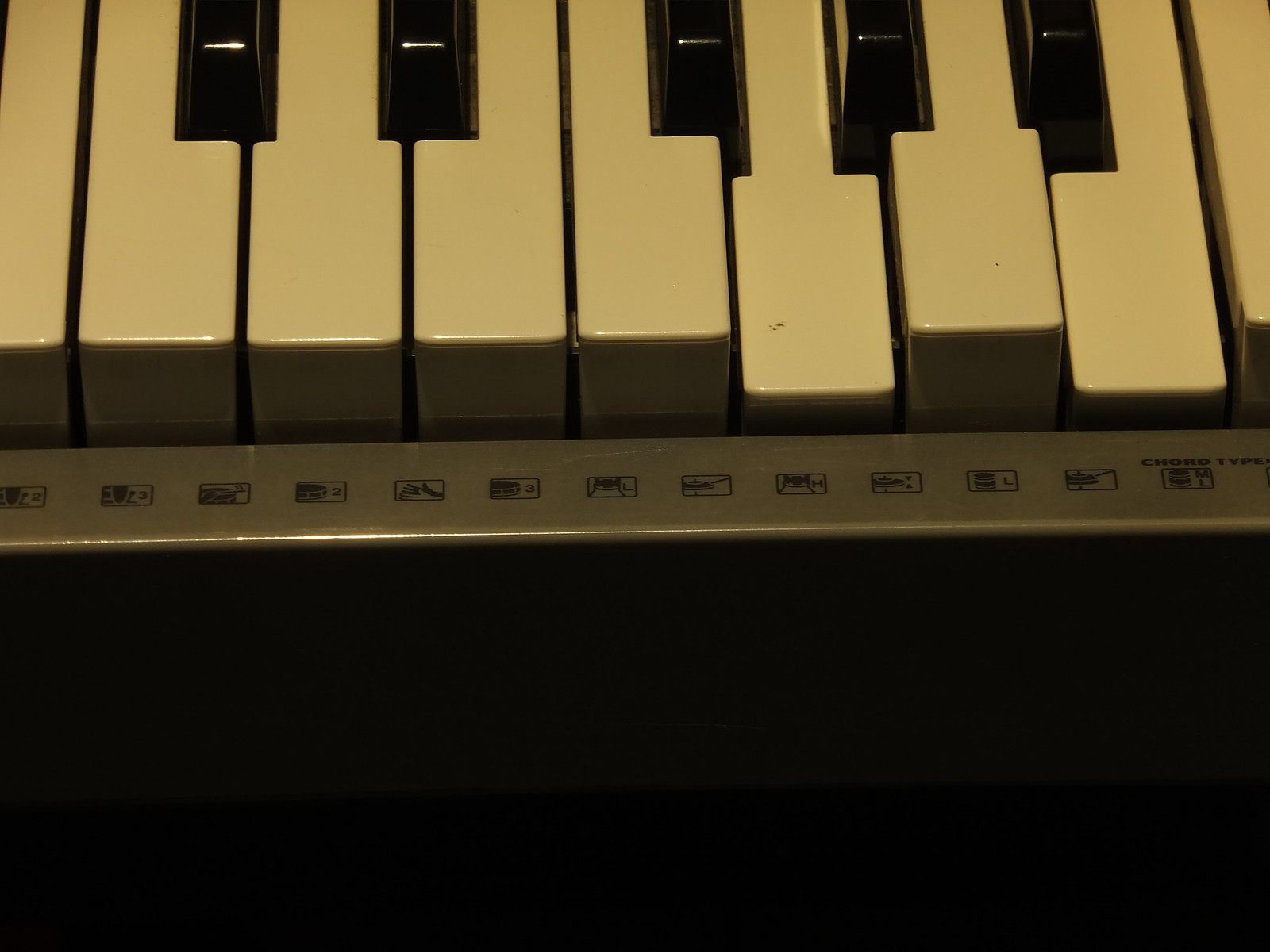This image is a close-up photograph of the bottom half of an electronic keyboard piano. The keyboard features nine white keys, with two of the white keys (the fifth and seventh from the left) being pressed down. We also see five black keys interspersed among the white ones. The keys have a yellowish tinge rather than a pure white color, indicating usage or age. Along the front edge of the keyboard is a silver bar with various little squares containing symbols or images. These include depictions of drum sticks, clapping hands, and chords, potentially providing cues or settings for different sound modes the keyboard can produce. The area beneath the keys is dark and not visible, adding to the focus on the keys and the symbol-laden silver bar.